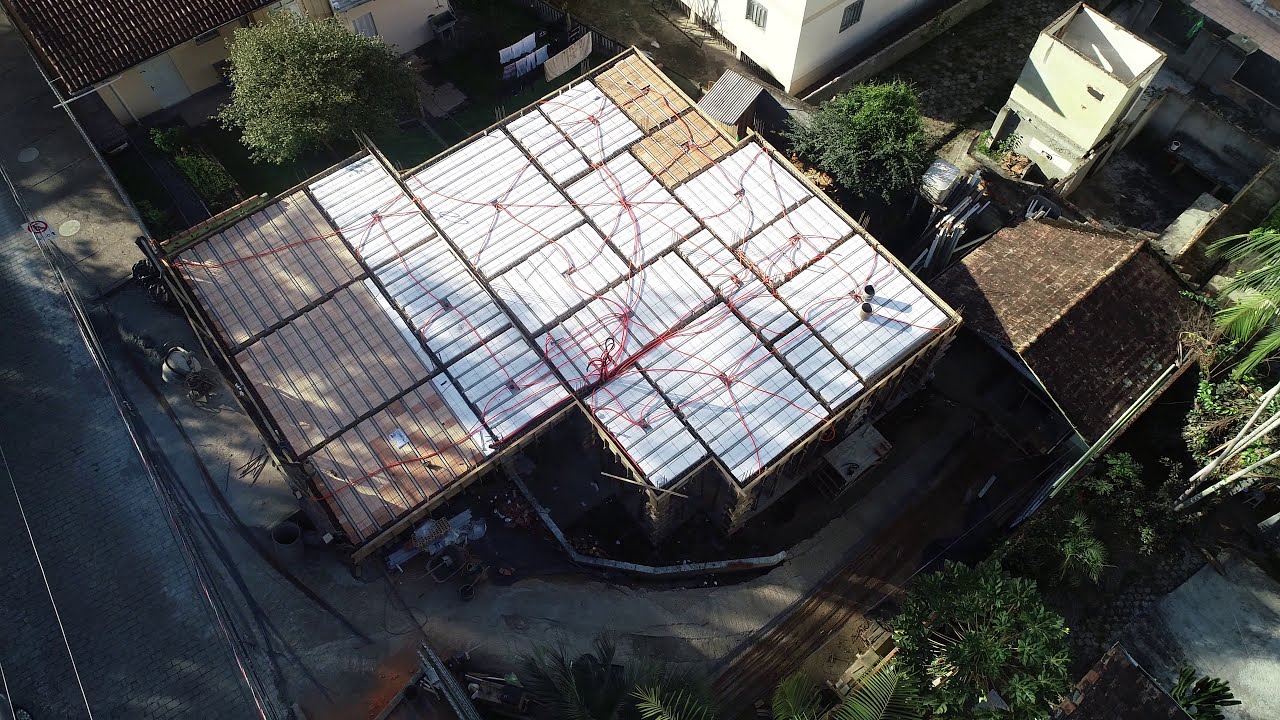This aerial photograph, likely taken by a drone, captures a detailed view of an urban neighborhood with the focal point being a centrally positioned modular building. The building's flat roof is segmented into various rectangular shapes of different sizes, connected by red wires that crisscross and converge at different points. To the left of this central structure, there is a series of three large modules, followed by smaller ones, and further spaced around are additional varied-sized rectangles, all interconnected by the red wires which were probably used for the building’s assembly.

Surrounding the modular building are other structures with distinct roofs, one of which is a regular home with a possible tile roof, alongside what could be a garage. There is a tree towards the top right corner of the image, suggesting the photo was taken in either spring or summer due to the greenery. The lower right side of the image also features additional trees. Encircling the central building, a road with gray asphalt runs along the left perimeter.

Overall, the atmosphere depicted is one of a bright sunny day, the sun’s position casting shades indicating a lower angle in the sky. The surrounding area includes pathways and possibly a small garden space directly below the main building, adding to the comprehensive urban landscape captured in this image.